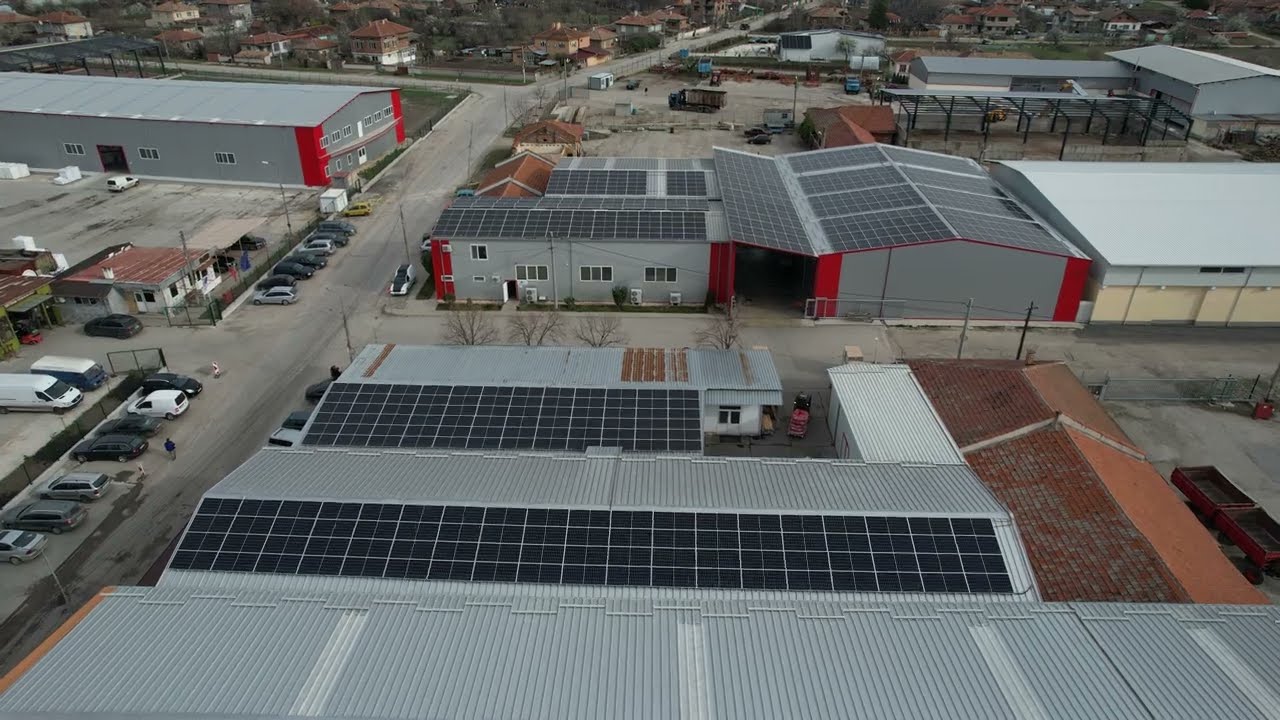This horizontal image showcases an expansive industrial and office complex characterized by numerous buildings with metallic gray roofs, many adorned with black solar panels. The structures exhibit occasional red accents along their edges and corners, adding a noticeable contrast. The scene is bustling with activity, evident from the plethora of cars parked in the extensive parking lots and streets lining the complex. On the left side of the image, a principal roadway runs seamlessly from the foreground to the background, flanked by parked cars and separated from the central buildings by silver fences. The road's continuation reveals an intersection further back, suggesting a connection to a distant town comprised of smaller houses and additional buildings. To the right, another street mirrors this layout, also populated with parked cars. The infrastructure, consisting mainly of large warehouse-like structures and office buildings, stretches out towards smaller buildings in the distance, all contributing to the intricate and detailed composition of this urban industrial landscape.